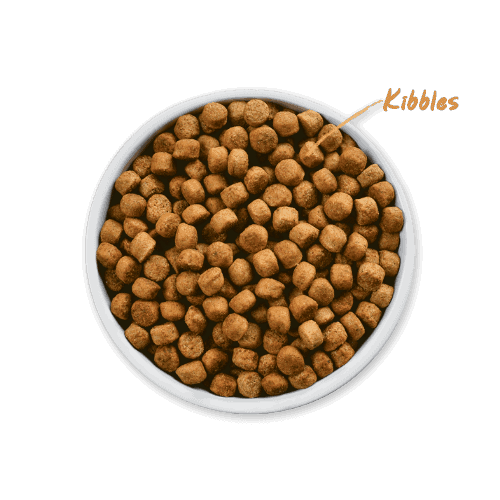The image features a centrally positioned, circular bowl set against a completely white background, creating an almost floating effect. The bowl, which appears to be made of either glass or plastic, displays a white rim. Inside the bowl are hundreds of small, rounded pieces of pet food, mostly dark brown interspersed with medium brown hues. The pieces are not perfectly circular but have rounded edges. At the upper right corner of the image, in brownish-gold italicized text, is the word "kibbles," with an arrow pointing towards the dog food. The detailed arrangement and setting give the impression that this could be a professional photograph for a pet food advertisement.